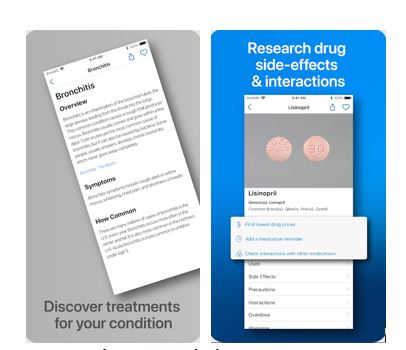Promotional Graphic for Health App Detailing Condition and Medication Information

The promotional graphic for a health-related app showcases two detailed screenshots, illustrating the app's user-friendly interface and comprehensive medical resources. 

In the left screenshot, the app provides an in-depth look at bronchitis, including an overview, symptoms, and prevalence. The bottom of the screen emphasizes the app's capability to help users discover treatments for their conditions.

The right screenshot focuses on the drug lisinopril, offering information on its interactions, side effects, prescriptions, and alternatives. Additionally, it features tools to find the lowest drug prices, add medications to a personal list, and check interactions with other drugs. Close-up images of the pill's front and back are also shown.

At the top of the graphic, a caption reads: "Research drug side effects and interactions," highlighting the app's purpose. Both images underscore the app's essential features, such as discovering treatments for various conditions and researching detailed drug information. This app aims to provide users with thorough and accessible medical knowledge.